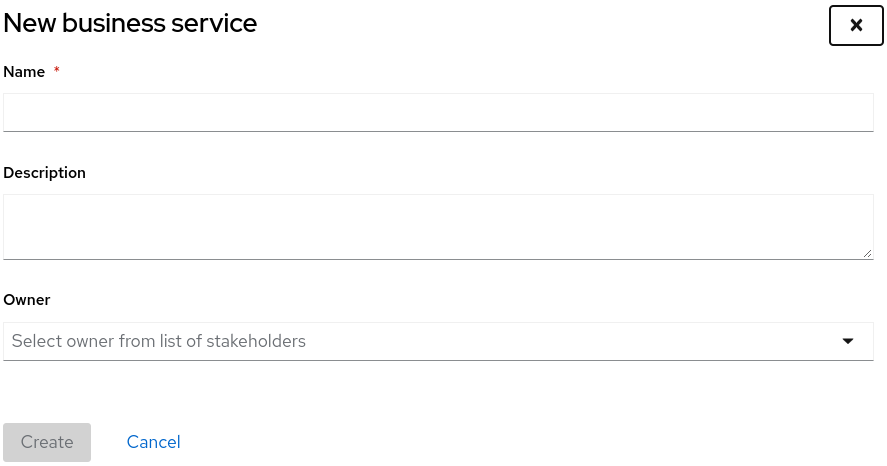The image displays a digital form for creating a new business service. At the top, in bold black letters, it reads "New Business Service." To the right-hand side of the page, there is a box with an "X" for closing the form. Below the heading, there's a field labeled "Name" followed by a red asterisk, indicating that it's a required field. Adjacent to this label is a blank line where users can input the name of the new business service. 

Following the "Name" field, there is a section labeled "Description." This section also includes a blank line where users can type a detailed description of the business service. Beneath the "Description" section, there is a label titled "Owner." Below this, the form instructs users to "Select owner from list of stakeholders," and it includes a drop-down menu indicated by a downward-facing arrow. 

Towards the bottom of the form, there are two buttons: a "Create" button located on the left, and a "Cancel" button in blue lettering on the right. The layout and instructions are clearly delineated to guide the user through the process of creating a new business service.